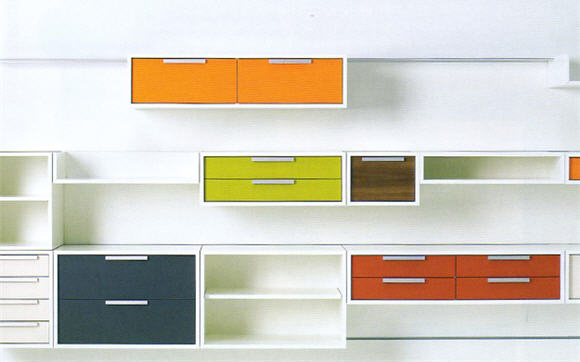The image depicts a modern, brightly colored shelving unit designed for an office, set against a white wall. The unit consists of multiple levels and a variety of drawers and shelves, giving it a cohesive yet dynamic appearance. 

At the top, there are two orange drawers encased in a white frame, mounted on a white track. Below this setup, to the right, are two white shelves and a series of four white drawers, all with silver handles, partially visible. The middle section features an eclectic mix—two tall, open white shelves stand beside two shorter yellowish-green drawers in a white cabinet frame. Adjacent to these is a smaller, square brown drawer, a white shelf, and a partial view of an orange drawer framed in white.

The bottom level showcases deeper blue drawers flanked by two sets of white and red drawers, each with four slim compartments. The unit is illuminated from the left side, creating a well-lit display that combines functionality and modern aesthetics seamlessly.